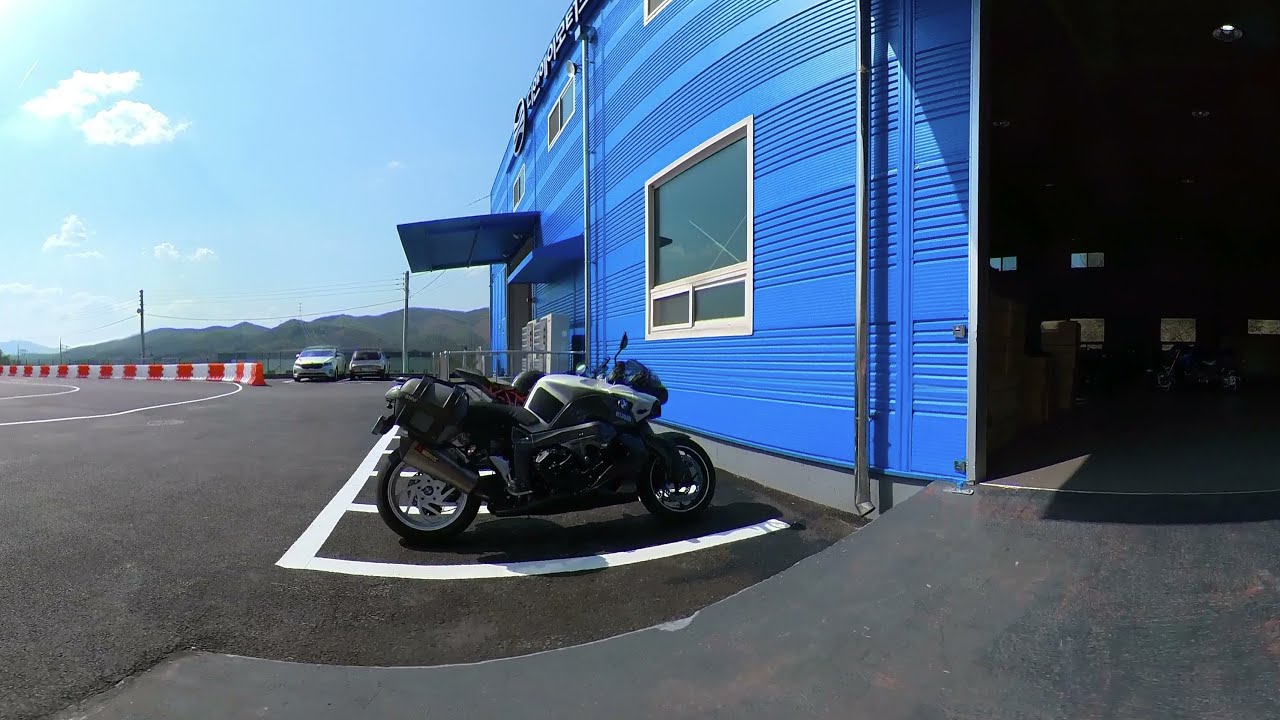A sleek, black and silver BMW motorcycle is parked in a reserved spot marked by white lines on a dark grey concrete surface, perfectly fitting its compact shape. This motorcycle faces an eye-catching bright blue building with a distinct, large window right beside it and a garage-like entrance to the right. The building features Korean text at the top center, adding an international flair. An orange and white dashed guardrail borders what appears to be a racetrack extending to the left behind the motorcycle. In the far background, you can see dark mountain ranges against a sky brushed with feathery white clouds. This outdoor scene captures a mix of elements, from the sleek motorcycle and the blue building’s silver awning to the expansive natural backdrop, suggesting a specialized garage facility adjacent to a racing track.